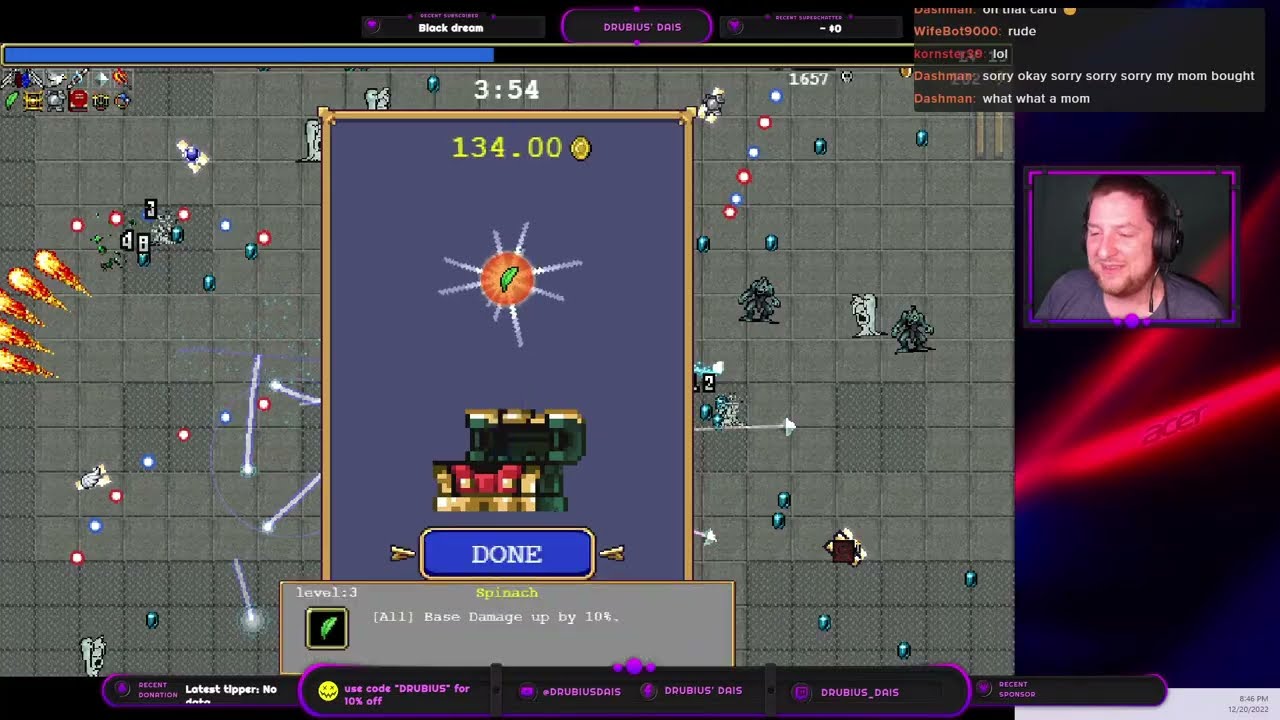The image is a detailed screenshot of someone streaming a video game. The background of the game is a gray grid pattern with lower quality images engaging in what appears to be a chaotic battle, with fireballs and laser beams. Dark and light characters are involved in the action. Amidst this chaos, a prominent purple screen with a gold edge overlays the game, displaying the amount $134.00 at the top. In the center of this screen, there is a green spinach leaf inside a red circle, accompanied by starburst effects.

Below the circle, there is a stack of books icon, and the text "Level 3 Spinach – All base damage up by 10%." A blue rectangle button saying "Done" is also visible. On the right side of the image, a man in his 40s or late 40s, wearing a scruffy beard, headset, and gray t-shirt, is seen streaming. He appears in a smaller purple box looking towards the game screen, which emphasizes his role in live commentary or interaction. Additionally, there are promotional phrases like "use code DRUBIOUS for 10% off" in the lower sections.